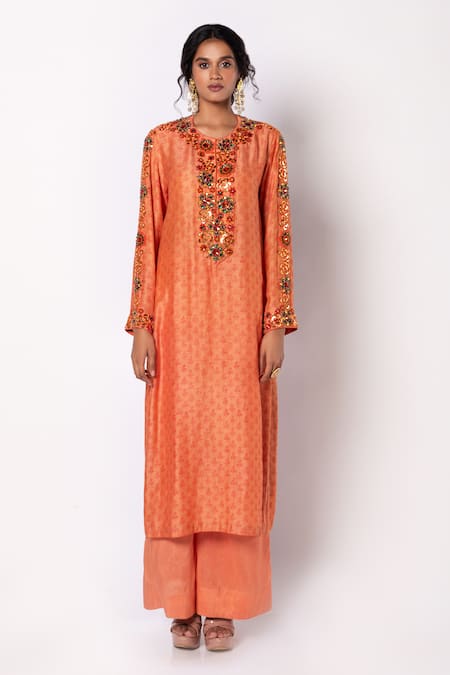A professional photograph features a woman standing in a formal, poised position. She is wearing a long, vibrant orange South Asian dress that reaches her ankles. The dress features elaborate colorful and floral patterns on the collar and long sleeves, and the upper part incorporates subtle patterned details within the orange fabric. The woman, likely a professional model, exudes a composed demeanor with her back perfectly straight and arms aligned straight down her sides. Adorning her dark, styled hair are long earrings that extend to her shoulders, adding to her elegant appearance. Set against a minimalist off-white background that might have a slight pink tint, the photograph is intentionally simple, drawing attention to the intricate details of her attire. A thin shadow of the woman is also visible on the plain backdrop, enhancing the professional quality of the image.